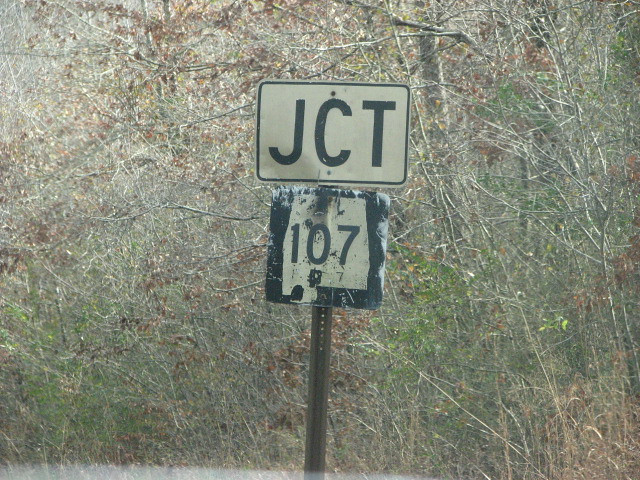This outdoor photograph captures a state road or route during late autumn, nearing winter. In the backdrop, there are bare trees with only a few remaining brown leaves, indicative of the season's transition. Prominently positioned in the foreground is a metal pole that rises from the bottom center of the image. This pole features small holes along its length and supports two signs at the top. The upper sign is a white rectangular plate displaying "JCT" in bold black letters, while the lower sign is black with a white outline of a state, containing the number "107."